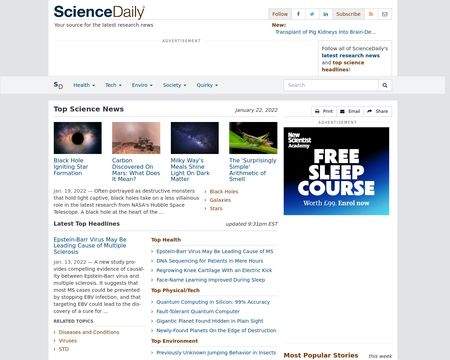In this image, we observe a screenshot set against a light lavender background, depicting the homepage of the website "Science Daily." At the top, there is a white rectangular banner featuring the site's name, with "Science" in bold black text and "Daily" in regular text, both indistinct due to the blurry view. The banner also carries the slightly blurred tagline: "Our source for the latest research news." On the upper-right corner, a light lavender button offers options to "Follow" and "Subscribe," accompanied by icons for Facebook, Twitter, and Instagram.

Directly below, a headline reads "New, transplant of pig kidneys," followed by a light lavender strip displaying the initials "SD." The site's navigation menu lists sections: Health, Tech, Enviro, Society, and Quirky, with a white search bar positioned to the right. Further down, a blue square with bold white text advertises a "Free Sleep Course."